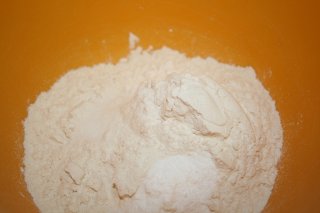The image showcases a bright orange-brown surface almost entirely covered in a pale, fine powder that closely resembles whole wheat flour. The flour covers most of the space, leaving only narrow borders on the left, right, and top edges. The powder forms a central pile with a peak, suggesting that some of it is sliding down the sides unevenly. The granules of flour are visible, with some forming larger, whitish chunks in the upper right-hand corner and another patch near the bottom. Tiny sprinkles of the powder are scattered at the top, as if they spilled out during pouring, adding to the overall textured appearance of the scene.